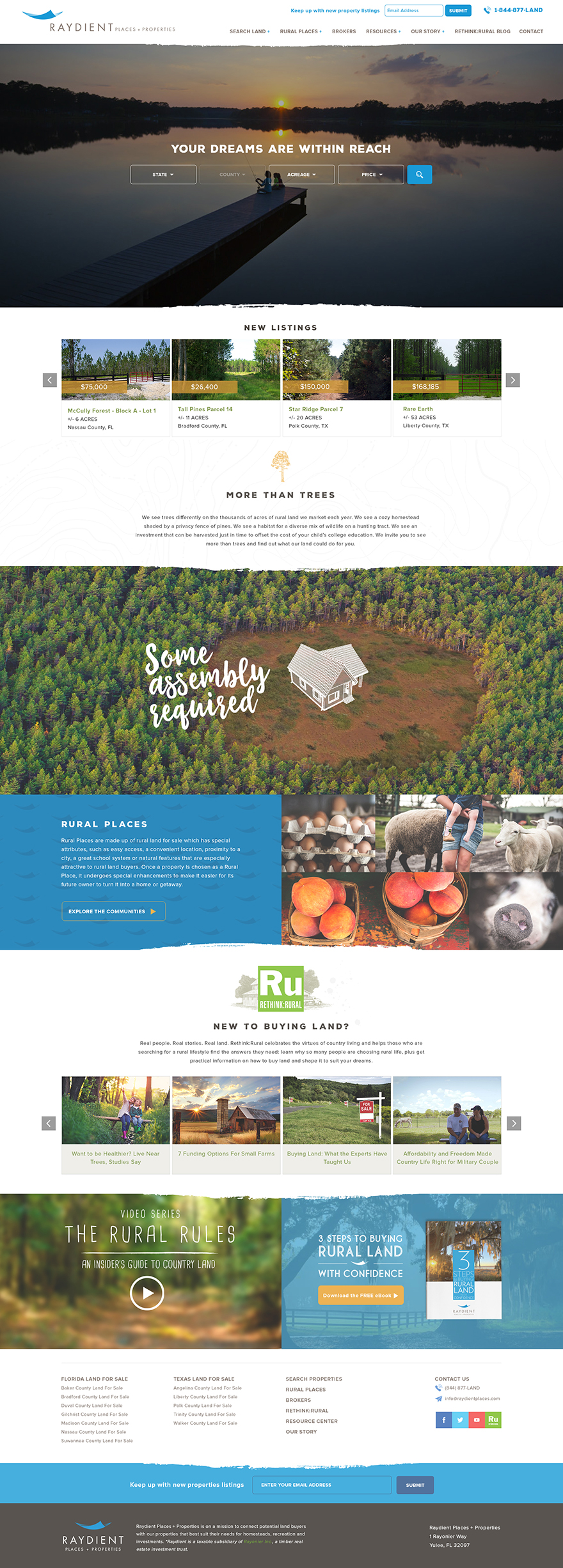Here's a detailed and cleaned-up descriptive caption for the image:

---

The screenshot captures a comprehensive view of a website. At the top, a blue logo is prominently featured on a white banner, complemented by black text and submenus. A blue and white search box is also visible at the upper section. As the viewer's gaze moves down, a captivating nature image emerges, depicting a sun setting over a serene body of water with a boat dock. People are sitting on this dock, enhancing the peaceful scene. Superimposed on the image is large, white text reading “Your dreams are within reach.” Below this, four boxes with white text are aligned horizontally.

Further down, a blue box is displayed, followed by a section featuring additional nature photographs. There are four images here, primarily showcasing green trees against a sky backdrop, accompanied by black text above. Continuing downward, an orange umbrella logo is noticeable, paired with black-font text and two paragraphs underneath it.

Another image appears below, boasting large white text that reads “Some assembly required.” This image shows a tan and gray farmhouse nestled in a field surrounded by trees. Adjacent to this is a blue box with white text. A series of farm-related images then follows, depicting eggs, sheep, and related scenes alongside a gray, white, and green logo and black-font text. Various additional images pop up, including photos of people and a “For Sale” sign.

Toward the bottom of the screenshot, more images are visible, of which one features trees while the other displays a mix of blue, orange, and white colors. The footer includes more text, submenus, and social media icons for Facebook and Twitter. Concluding the webpage is a blue banner with white text, followed by a gray banner that contains both white and blue text.

---